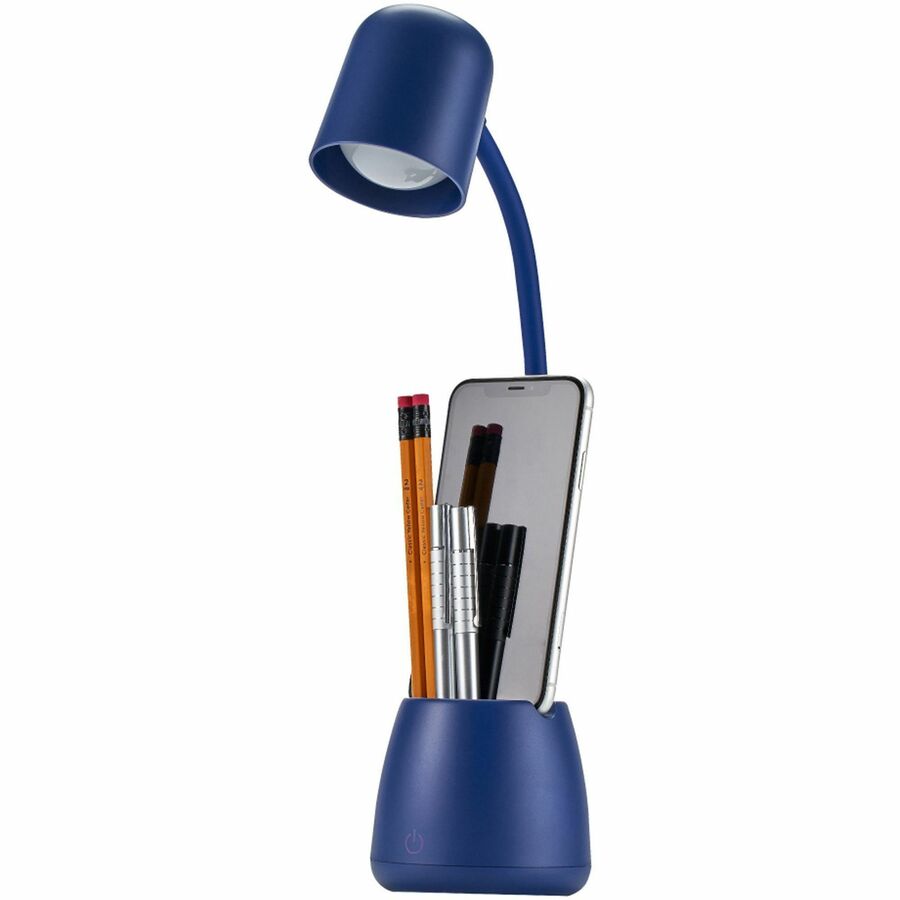The desktop lamp has a multi-functional, modern design, ideal for student use and crafted to save space. The lamp features a navy blue, cup-like base that serves as a pencil holder, with an open notch that securely holds a smartphone. The base contains several writing utensils, including two yellow pencils, two silver pens, and two black pens. The smartphone nestled in the notch reflects these utensils. The thin neck of the lamp extends upward to a smaller, similarly navy blue lampshade that houses a prominent white bulb. An intuitive on/off button, resembling a digital emblem, is situated on the base, simplifying operation. The overall look is sleek and minimalistic, designed to fit seamlessly on any desk.